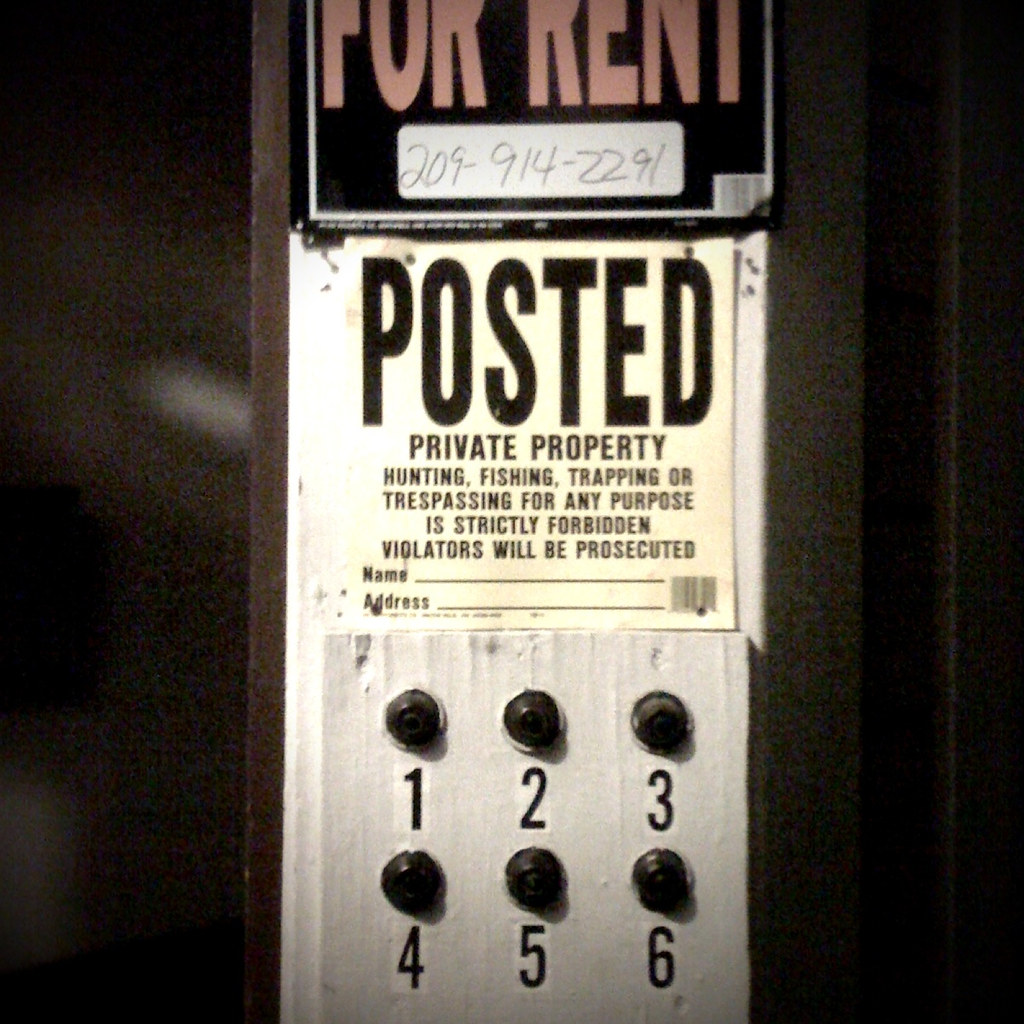This image depicts the detail-rich panel potentially inside or adjacent to an elevator. At the top of the panel, there is a black sign with red text that reads "For Rent" and a contact number, "2099142291," displayed in a white bar at the bottom of the sign. Below this, a white sign with bold black text prominently features the word "Posted," followed by smaller text clarifying that it is Private Property. The sign firmly states: "Hunting, Fishing, Trapping, or Trespassing for any purpose is strictly forbidden. Violators will be prosecuted." There are fields labeled for a name and address, but both are left blank. Below these signs, the panel includes two rows of black buttons labeled with numbers, where the top row comprises buttons numbered 1 to 3, and the bottom row 4 to 6.